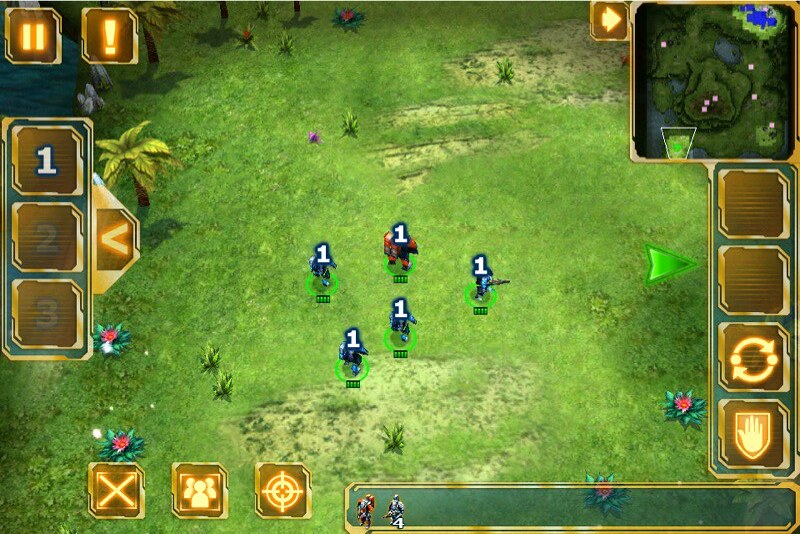This image is a detailed screenshot from a video game, featuring a cartoony, computer graphic representation of a green field viewed from an overhead perspective, reminiscent of a battle scene. Dominating the center of the screen are five small avatars, each marked with a white number one, outlined in blue, and encircled by green rings. These numbers and rings partially obscure the avatars. The field itself has patches of brown, random plants, and a couple of palm trees adding to its texture.

In the upper right corner, there's an inset map providing an overview of the field. Adjacent to this inset are toggles, including a replay button and a stop button. The left side of the screen features a vertical arrangement of numbers one, two, and three, with the number one highlighted. Below this, in the bottom left corner, there are three blocks with unique designs: one with an X, another resembling flower petals, and the last depicting a target. Scattered throughout the field are items such as arrows and coins, adding to the game's interactive elements. Additionally, menu buttons and what appears to be a chat bar are situated at the bottom right of the screen, completing the interface.